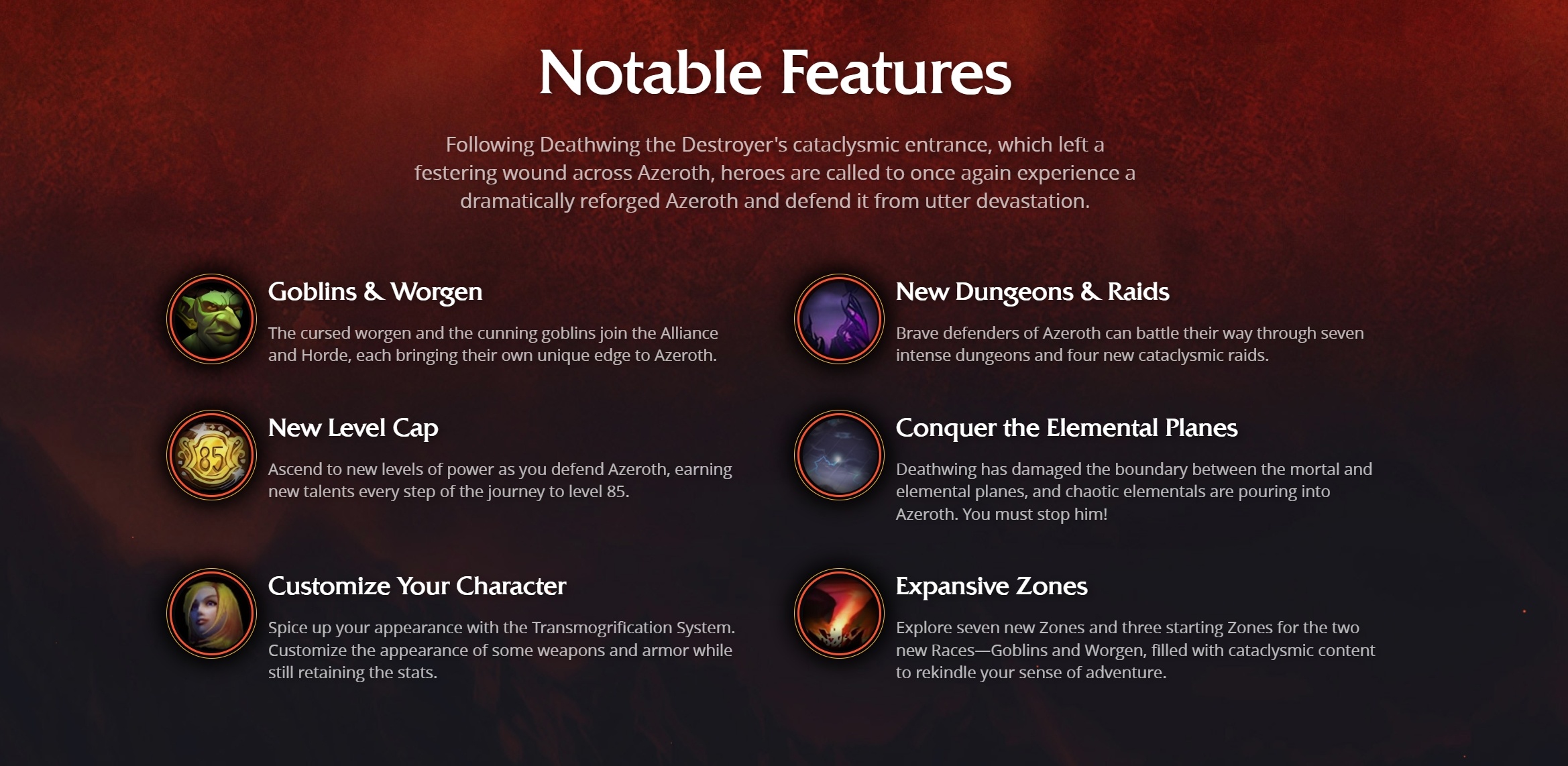The image is a crimson red or burgundy rectangular infographic highlighting notable features of a video game, likely World of Warcraft. At the top, the headline "Notable Features" is prominently displayed in large white letters. Below this, a brief paragraph in white text reads, "Following Deathwing the Destroyer's cataclysmic entrance, which left a festering wound across Azeroth, heroes are called to once again experience a dramatically reforged Azeroth and defend it from utter devastation."

On both the left and right sides of the rectangle, there are six red circles, each containing a character or scene along with labels and a short description in small white text. The labels read: 
1. "Goblins and Worgen" - displaying a green Goblin icon, highlighting, "The Cursed Worgen and the Cunning Goblins join the alliance and horde, each bringing their own unique edge to Azeroth."
2. "New Level Cap" - detailing the path to level 85 with, "Ascend to new levels of power as you defend Azeroth, earning new talents every step of the journey."
3. "Customize Your Character" - emphasizing character customization options.
4. "Dungeons and Raids" - focusing on new dungeons and raid experiences.
5. "Conquer the Elemental Plains" - portraying a fiery scene.
6. "Expansive Zones" - showcasing the broad new areas to explore.

Each bullet point has a corresponding red circle icon with one or two descriptive sentences, enhancing the rundown of the game’s exciting new features.